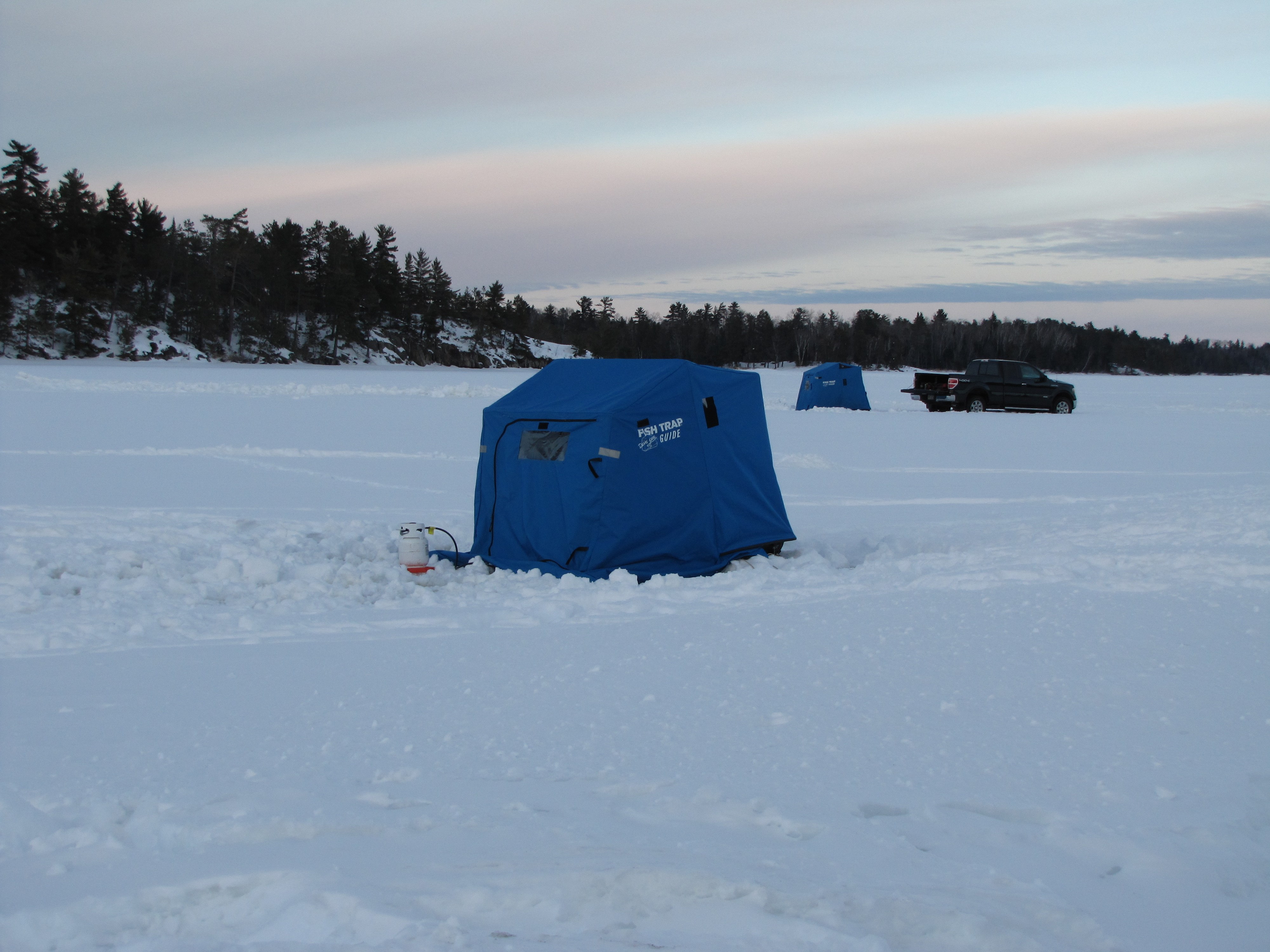In this photographic image taken outdoors on a frozen lake during the day, we see a serene winter scene. The background features a gray-blue sky with white and pink clouds, suggesting either early morning or late evening light. Silhouetted against the sky is a stand of trees, creating a stark contrast with the snowy landscape below.

The foreground is covered with a pristine field of snow, indicative of the iced-over lake. Dominating the center of the photo is a medium blue tent, likely a fishing shanty, with white lettering stating "Fish Trap" on a black label sewn onto it. Attached to the back of the tent is a canister of LP gas. Just behind this tent, there is another similar blue tent and to the right of these tents, there is a parked pickup truck with its tailgate open. The overall atmosphere suggests a tranquil ice fishing expedition.